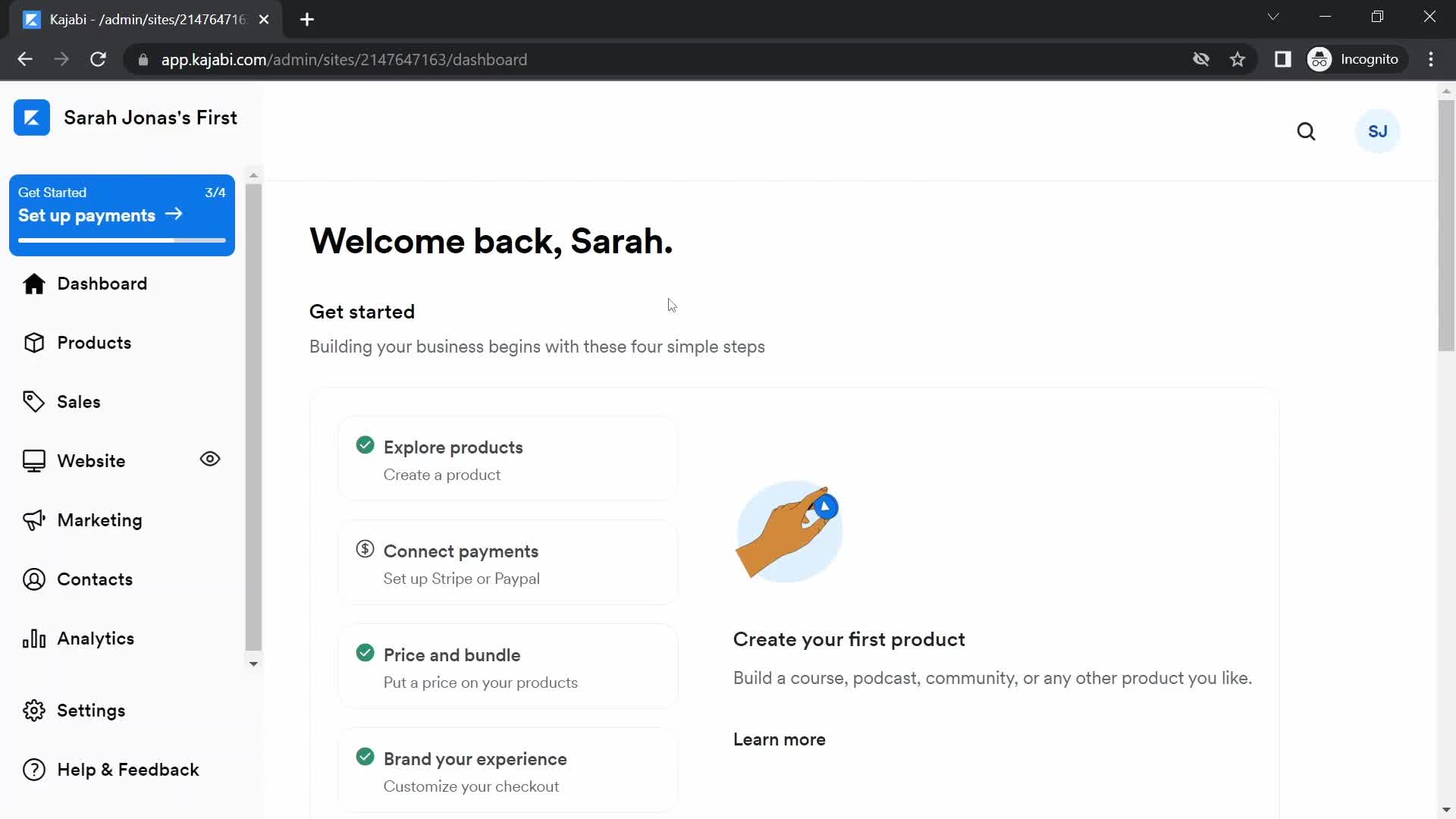In this image, we observe a screenshot displaying a computer screen with an incognito browser tab open. The website interface features a prominent header in the upper left-hand corner that reads "Sarah Jonas." Below this, along the left-hand sidebar, are various navigational options including "Get Started," "Set Up Payments," followed by buttons for "Dashboard," "Products," "Sales," "Website," "Marketing," "Contacts," "Analytics," "Settings," "Help," and "Feedback."

The central portion of the screen presents a personalized welcome message: "Welcome Back, Sarah." Below this greeting, the screen directs users to begin building their business with four outlined steps: "Explore Products," "Connect Payments," "Price and Bundle," and "Brand Your Experience." 

To the right of these steps, additional options encourage Sarah to "Create Your First Product" which could be a "Course," "Podcast," "Community," or any other product she prefers. A "Learn More" button is positioned on the far right side of the screen.

A gray scroll bar is visible at the very top of the window. Additionally, a profile icon featuring the initials "SJ" is located in the upper right corner, indicating Sarah's profile section.